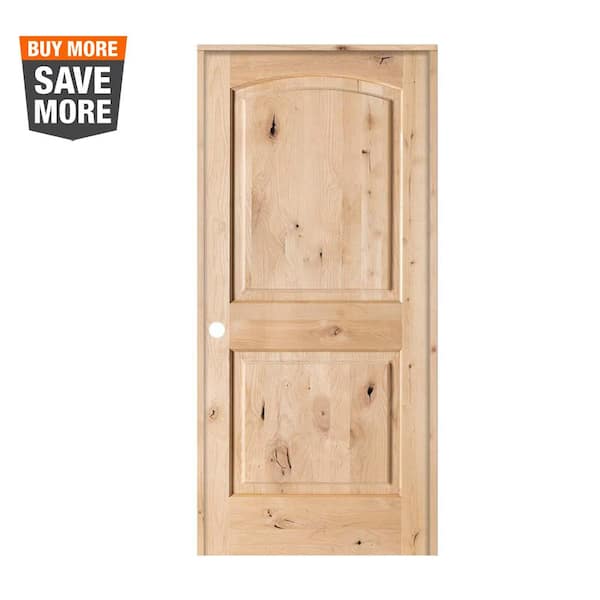The image depicts an unfinished light brown wooden door that could potentially function as a front door, pantry door, closet door, or bedroom door. The door is crafted from light wood, possibly cedar, featuring visible wood grain and knots throughout its surface, with seven knots in the top panel and six in the bottom panel. The structure of the door includes two main panels with a rim around the edges. The top panel is rectangular with a rounded top, while the bottom panel is a simple square. A round hole for a doorknob is located on the left side, slightly below the middle. The door is set against a white background. In the upper left-hand corner of the image, there is a black and orange shield-shaped geometric figure. The top part of the shape holds white letters on an orange background that reads "buy more," and the bottom part, in white letters on a dark gray background, says "save more."